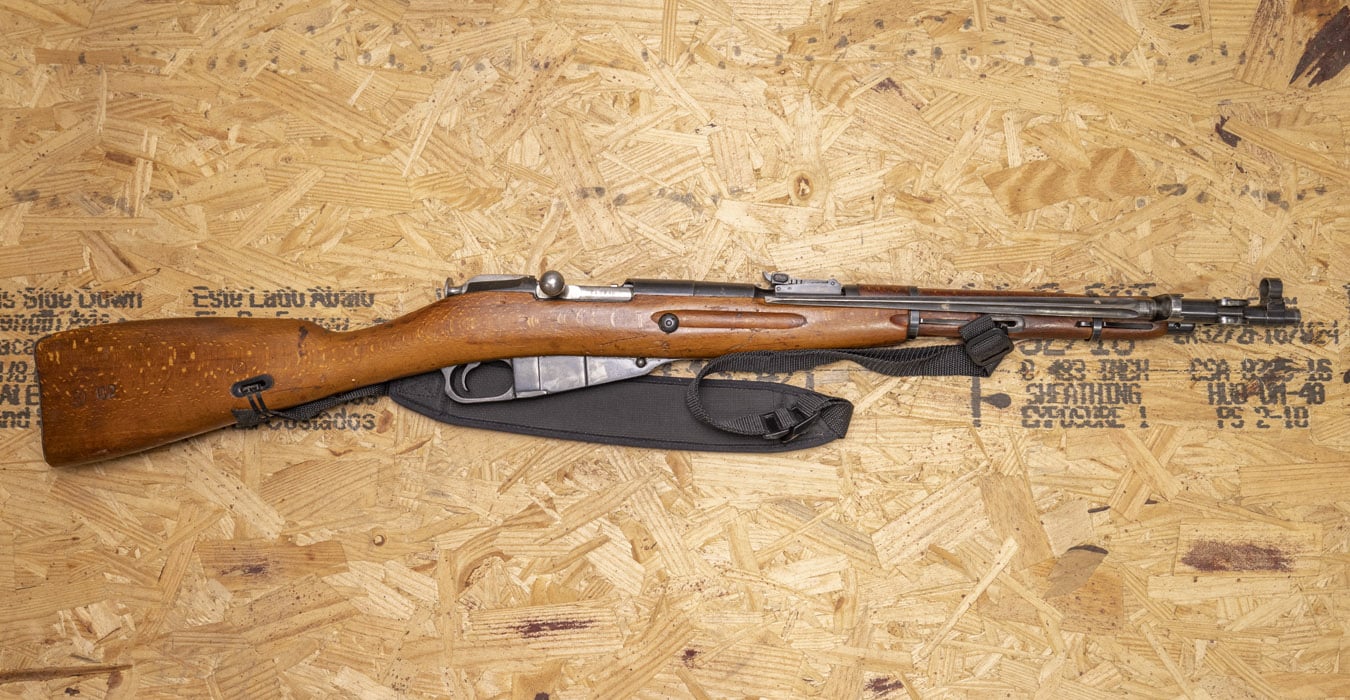The image depicts an aged rifle, likely a single-shot, bolt-action type, lying flat and displayed on what appears to be a light brown, pressed plywood platform, which is likely mounted on a wall. The plywood bears black text, which is partially obscured and faded, making it hard to read clearly. The rifle features a brown body with a dark brown handle positioned on the left side of the image, and the barrel includes both wood and black gunmetal components. The buttstock of the rifle is also brown, speckled with white. Below the dark silver trigger, a black strap is attached, looping towards the base of the rifle. The tip of the barrel has a sighting hole for aiming. The rifle appears to be well-worn and possibly held in place by nails or hooks driven into the plywood.